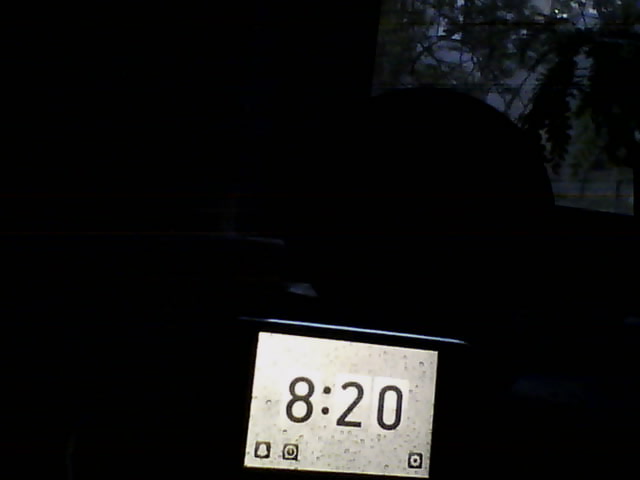This square-shaped image predominantly features a digital screen located centrally at the bottom. The screen is rectangular with a white background and displays the time "8:20" in black font. Surrounding the time display are several black dots scattered across the background. In the bottom-left corner, there’s a notification symbol resembling a bell, and to the bottom-right, there is a clock icon. The rest of the image is quite dark and blurry, compromising its overall quality.